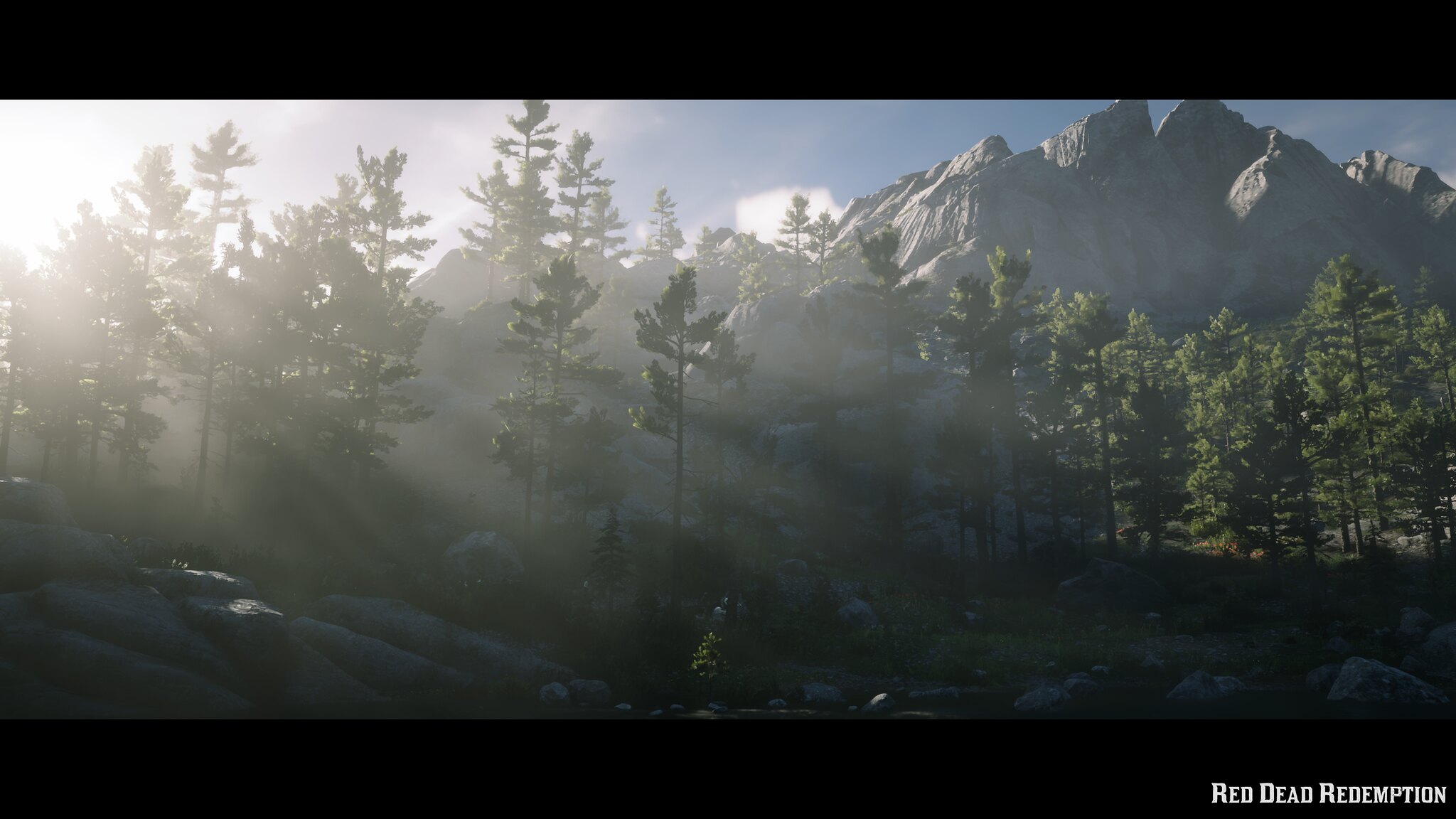In this stunning image from the game Red Dead Redemption, the viewer is treated to a breathtaking vista of the vast wilderness. The bottom right-hand corner of the image confirms the game's title with white text, ensuring there's no mistaking the origin of this remarkable scene. The foreground is dominated by a lush forest, with a variety of trees at different heights, some taller than others due to the undulating terrain. These trees are bursting with green leaves, suggesting a vibrant spring or summer season, and the ground below is carpeted with verdant grass.

Beyond the forest, a massive mountain looms, its jagged edges starkly etched against the sky. The sun beams down from above, casting radiant shafts of light through the tree branches, creating a mesmerizing interplay of light and shadow. The mountain slopes are steep and dramatic, and the highest peaks stand bare, devoid of any tree cover, accentuating their towering, unyielding nature. This detailed depiction immerses the viewer in the game's rich, natural environment, highlighting its serene yet majestic landscape.